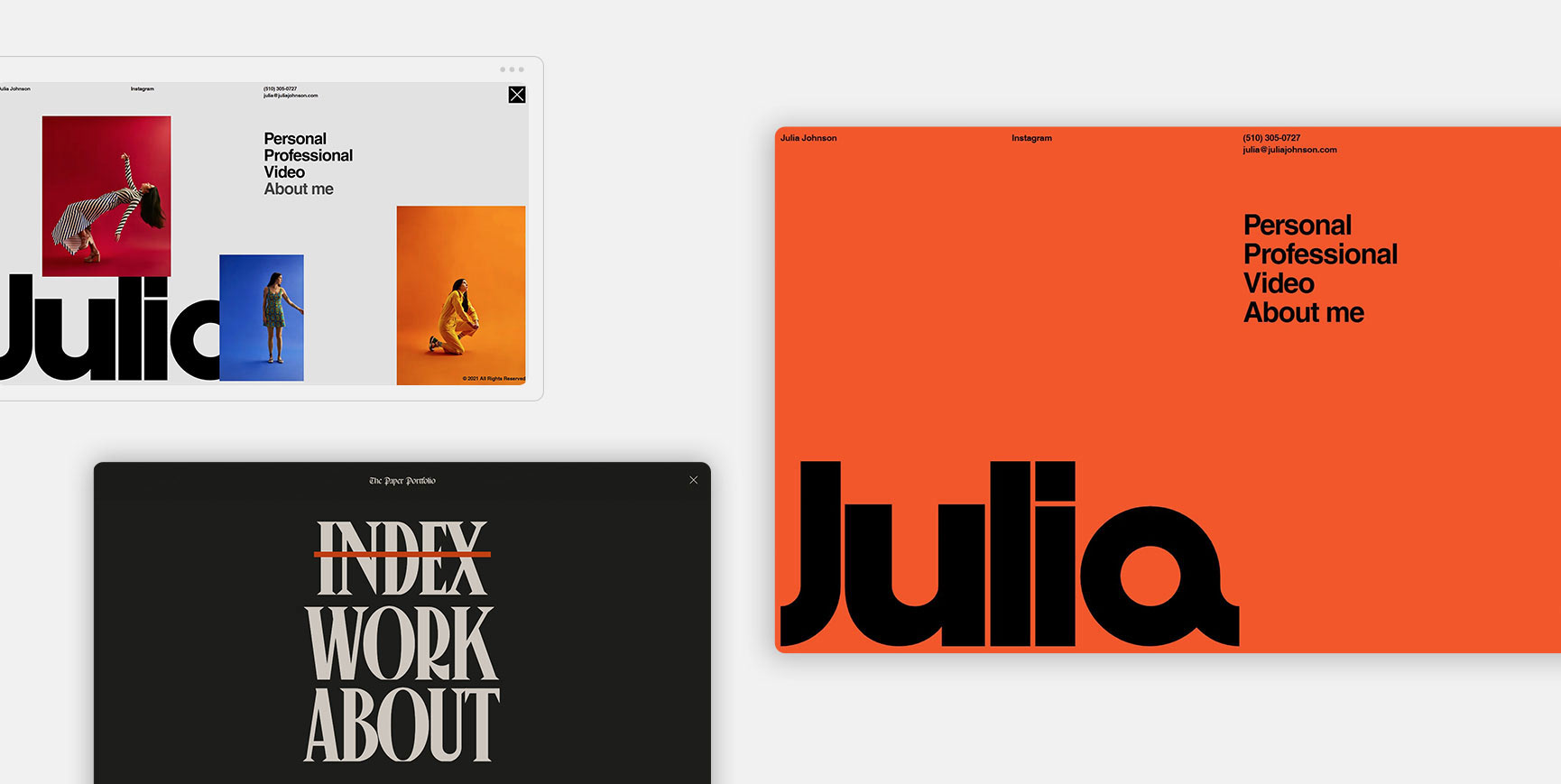The image displays a detailed digital webpage layout with three distinct sections, all set against a clear, white background. The top left section showcases three photos of women, labeled "personal," "professional," and "video about me," with the name "Julia" in black letters at the bottom left corner. Each woman's photo contrasts with a different background color—red, blue, and orange, respectively. The woman in the red background wears a white and black striped gown and poses bending backwards with open black hair. The woman against the blue background is clad in a green sleeveless mini skirt, while the woman in the orange background sports a yellow jumpsuit and kneels on the ground.

Directly below this, there’s a black background section with the title "index" crossed out in red, alongside the words "work" and "about" in white letters. The top right-hand corner of this section features a close icon. Overlaying the image are social media icons and contact details including an Instagram logo and a phone number, (510) 305-0727, plus an email address: julie@juliejohnson.com. A footnote reads "copyright 2021 all rights reserved."

On the right-hand side of the overall layout, an orange background page repeats the name “Julia” along with the captions "personal," "professional," and "video about me" in black letters, accompanied by the same contact information including Instagram, phone number, and email. This segment further emphasizes the cohesive brand identity with its use of consistent details and formats.